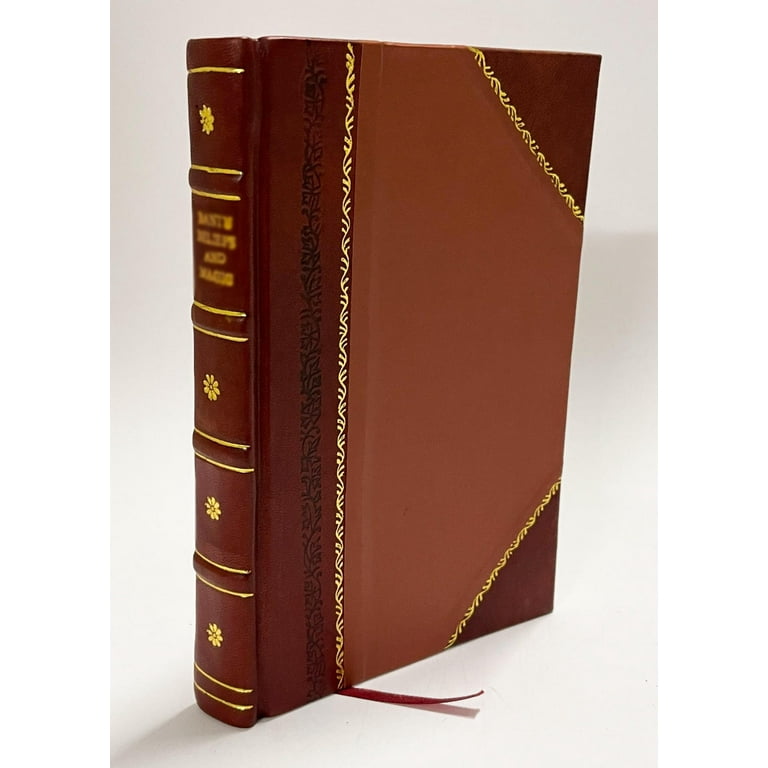This image captures an elegantly ornamental, leather-bound book standing upright as if on a bookshelf. The background is a solid light gray, which highlights the book's intricate design. The book’s binding, in a deep red hue, is adorned with squares running down the spine, featuring delicate gold flower icons—one per square—with a blurred-out title located near the top. The front cover showcases a beautifully intricate pattern: the deep orange central panel is framed by red corners with thin gold vines outlining them, and a striking black vine running vertically along the binding, paralleled by a slimmer gold vine. Extending from the bottom of the book is a brown ribbon bookmark. The overall condition of the book is excellent, suggesting it is well-preserved despite its age.